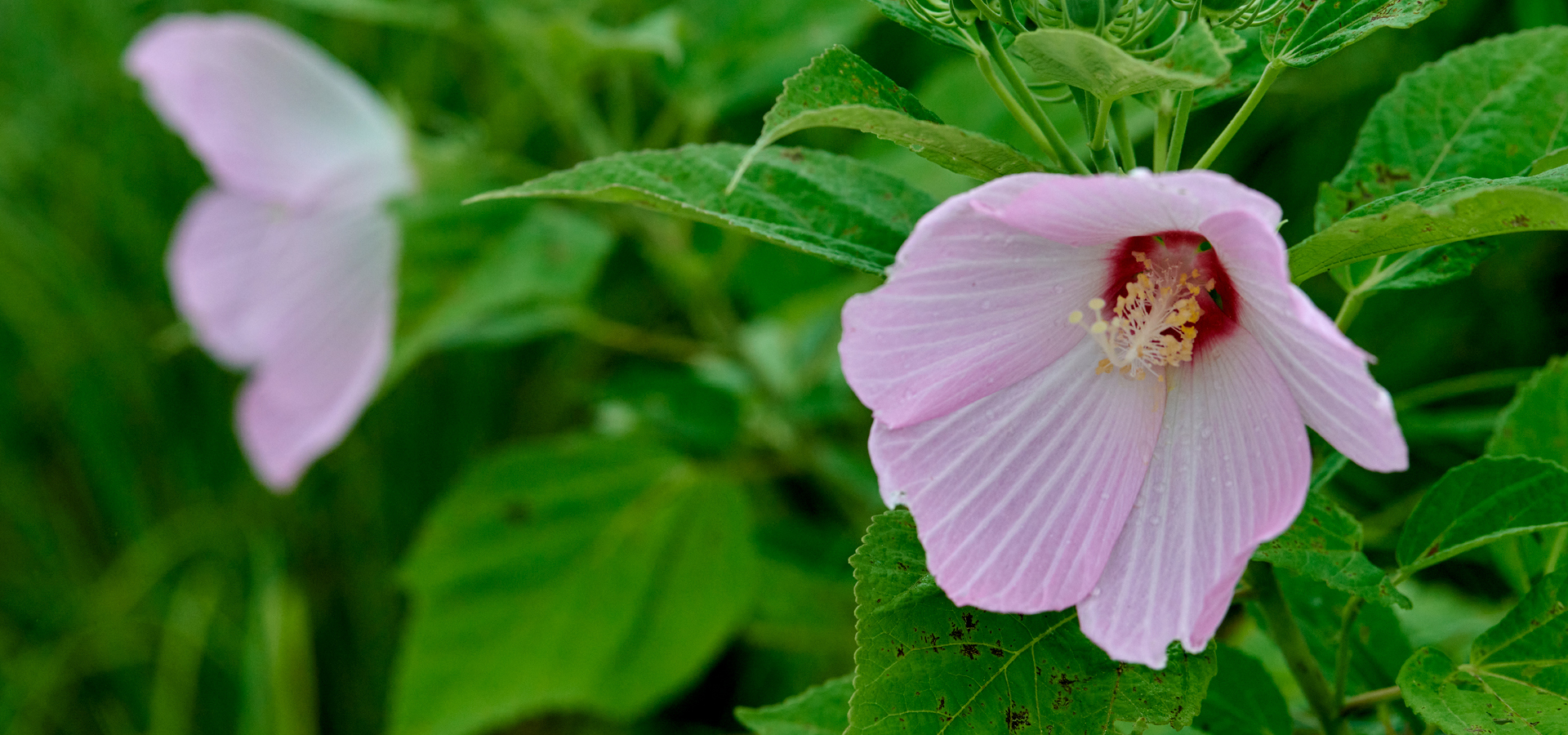This horizontal rectangular photograph captures the striking beauty of a tropical pink flower, likely a hibiscus or lily, set against a vibrant green backdrop. The focus of the image is a single, stunning bloom positioned in the right third of the frame. This flower features delicate petals with a red blush at the center, gracefully leading to a prominent yellow pollen structure that extends outward. The petals display a spectrum of soft whites blending seamlessly into the vibrant pink, adding depth and texture to the flower's appearance. Surrounding the flower are bright green leaves, notable for their healthy glow but with small, worn specks that hint at natural wear and tear. In the background, blurred almost to abstraction, is another pink flower, providing a subtle contrast without diverting attention from the main subject. The shallow depth of field creates a dreamy, soft-focus effect, enhancing the overall tropical and serene ambiance of the scene.